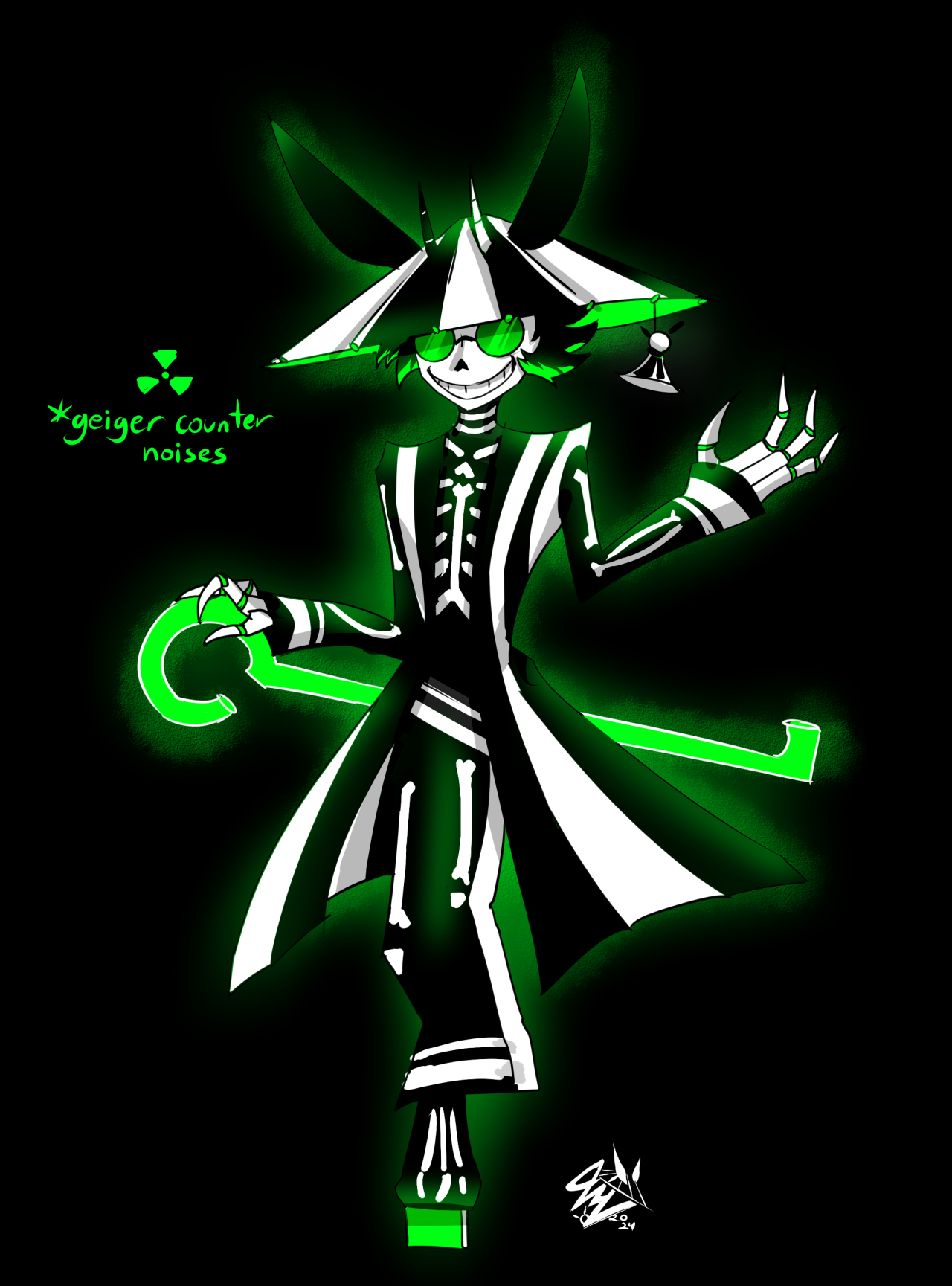The image is a tall, rectangular digital artwork set against a completely black background. At its center is a character that merges elements of a skeleton and a robot. Its head, positioned just below the top of the image, is white with black and green spiky hair. The character dons a dome-shaped hat with two dark green, bunny-like ears and an East Asian conical style featuring black and white gradients. This psychedelic figure sports green sunglasses and has a jack-o'-lantern type smile. Its outfit consists of a long, black and white striped trench coat that flares out at the bottom, complemented by matching pants. The character’s silver hands, highlighted with green at the hinges, hold a large, glowing green key behind its back. To the left, in green font, the caption reads "Geiger counter noises."